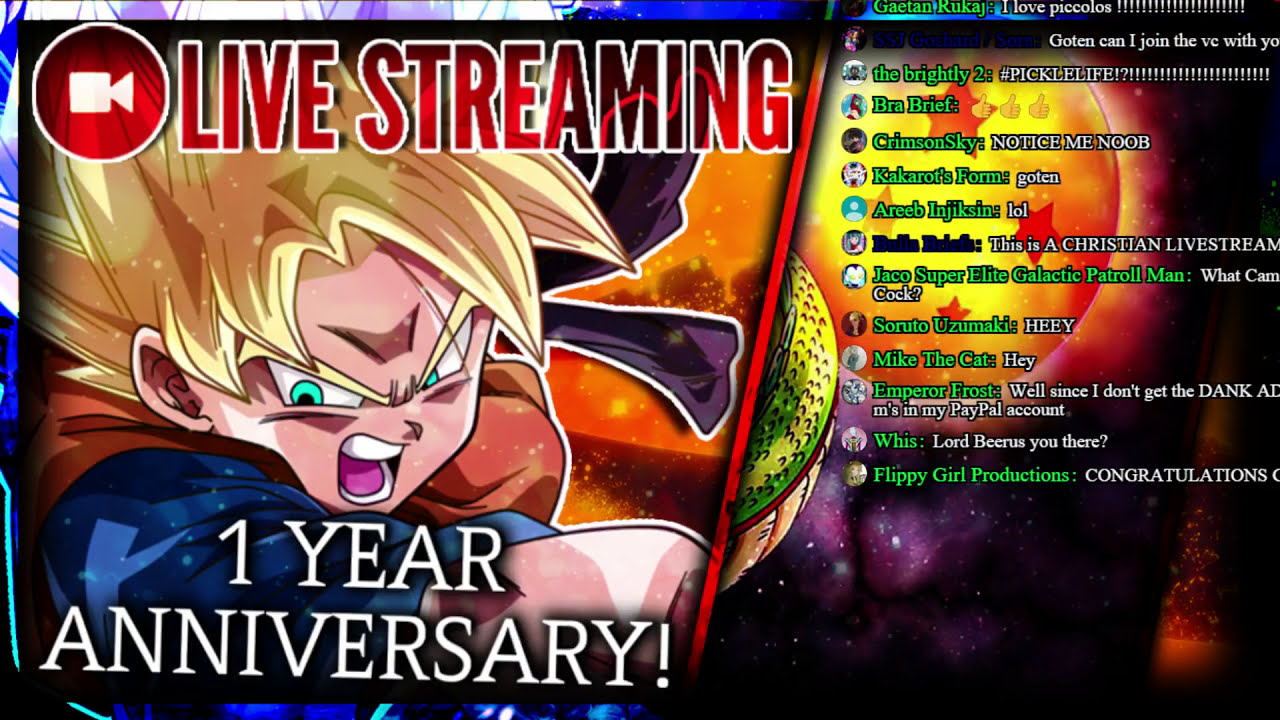The image is a vibrant and colorful screenshot of a live streaming event celebrating its one-year anniversary. On the left side of the image, there is a striking depiction of a male anime character who appears to be from Dragon Ball Z, possibly Goku. He has spiky blonde hair, intense green eyes, and an angry expression as if he is in the middle of a battle. He is dressed in a blue and orange outfit with flashes of purple. Above the character, in bold red letters, it says "Live Streaming" accompanied by a red recording icon, and below in white letters, it reads "One Year Anniversary." The background of the image is a space-like atmosphere with shades of black and purple, dotted with tiny white stars, and a prominent bright sun-like object in the top right corner, radiating orange and yellow with reddish-orange stars. A red bar segments the chat section from the main image. The live chat on the right features various messages from viewers, with names appearing in green and messages in white. Comments include phrases like "pickle live," "notice me noob," "gotten lol," and "this is a Christian live stream," among others, highlighting the interactive engagement of the audience.